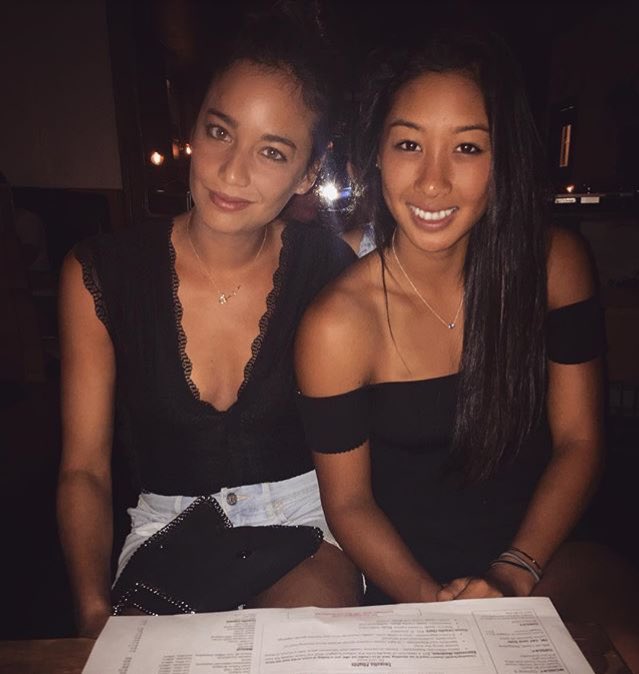In the dimly lit ambiance of a quiet restaurant, two women are prominently featured in the center of the image, positioned perfectly side by side. Both women are dressed in black dresses, suggesting a coordinated or formal outing. The woman on the left has her dark hair pulled back and is adorned with a black dress featuring a low-cut, lace-adorned v-neckline that extends to lace detailing on the shoulders. Around her waist, she wears white shorts or possibly a white belt or jacket, and she may also have a black purse or linen napkin on her lap. Her head is slightly tilted towards the woman on the right, and she smiles softly with dark eyes and pronounced eyebrows.

The woman on the right, with her long, thick, dark hair cascading past her chest, wears an off-the-shoulder black dress, showcasing her bracelets. She has a broader smile and dark eyes, reflecting a sense of warmth and camaraderie. Both women are seated at a table, evident from the menu positioned at the bottom of the screen. Behind them, a mirror reflects other guests, hinting at the sociable atmosphere of the restaurant. The color palette of the image consists of various shades of white, black, brown, tan, and yellow, adding to the cozy yet chic environment.